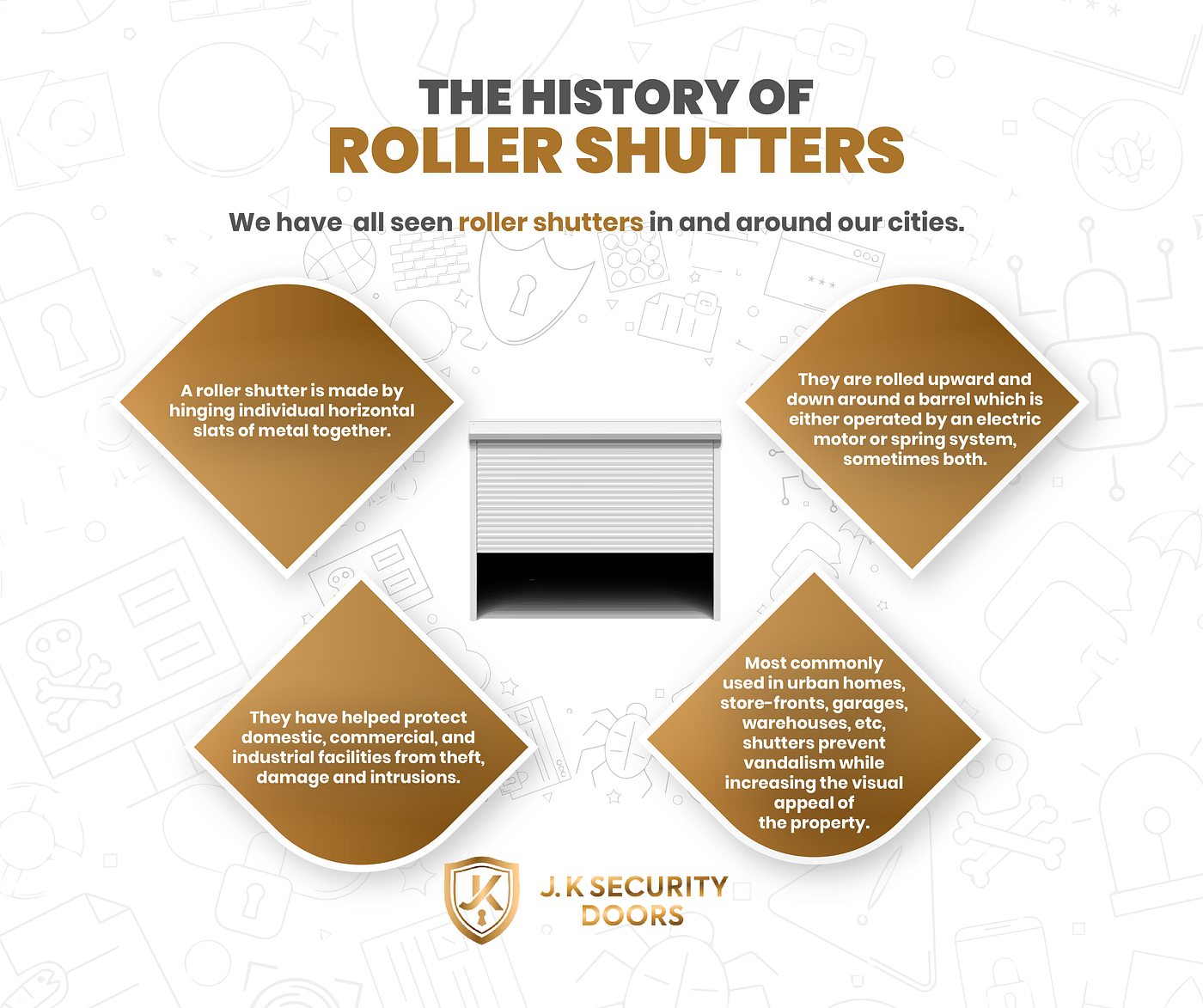This marketing poster, set against a white background faintly adorned with sketches of badges, locks, and circles, intricately details the history and prevalence of roller shutters. The top of the poster features a title in black, uppercase text reading "The History of." Below, in slightly larger brown uppercase letters, it states, "Roller Shutters." Following this, in smaller black letters, the text reads, "We have all seen roller shutters," with "roller shutters" highlighted again in brown, "in and around our cities."

Centrally placed is a black-and-white photograph depicting a half-open roller shutter door, typically seen over shop entrances. This visual anchors the design, its lower part shadowed in dark gray while the upper part features the rolled-up shutter.

Surrounding the photograph are four brown diamond-shaped callouts with curved tops, each outlined in white and inscribed with white text. These callouts, positioned to the upper left, upper right, bottom left, and bottom right of the photograph, likely describe various historical aspects and features of roller shutters, although the text is too small to read clearly.

At the very bottom of the poster, in the center, is a shield symbol with the letters "JK" inside, next to the text "JK SECURITY" in goldish-brown letters, with the word "DOORS" directly beneath it. This logo solidifies the brand presence of JK Security Doors.